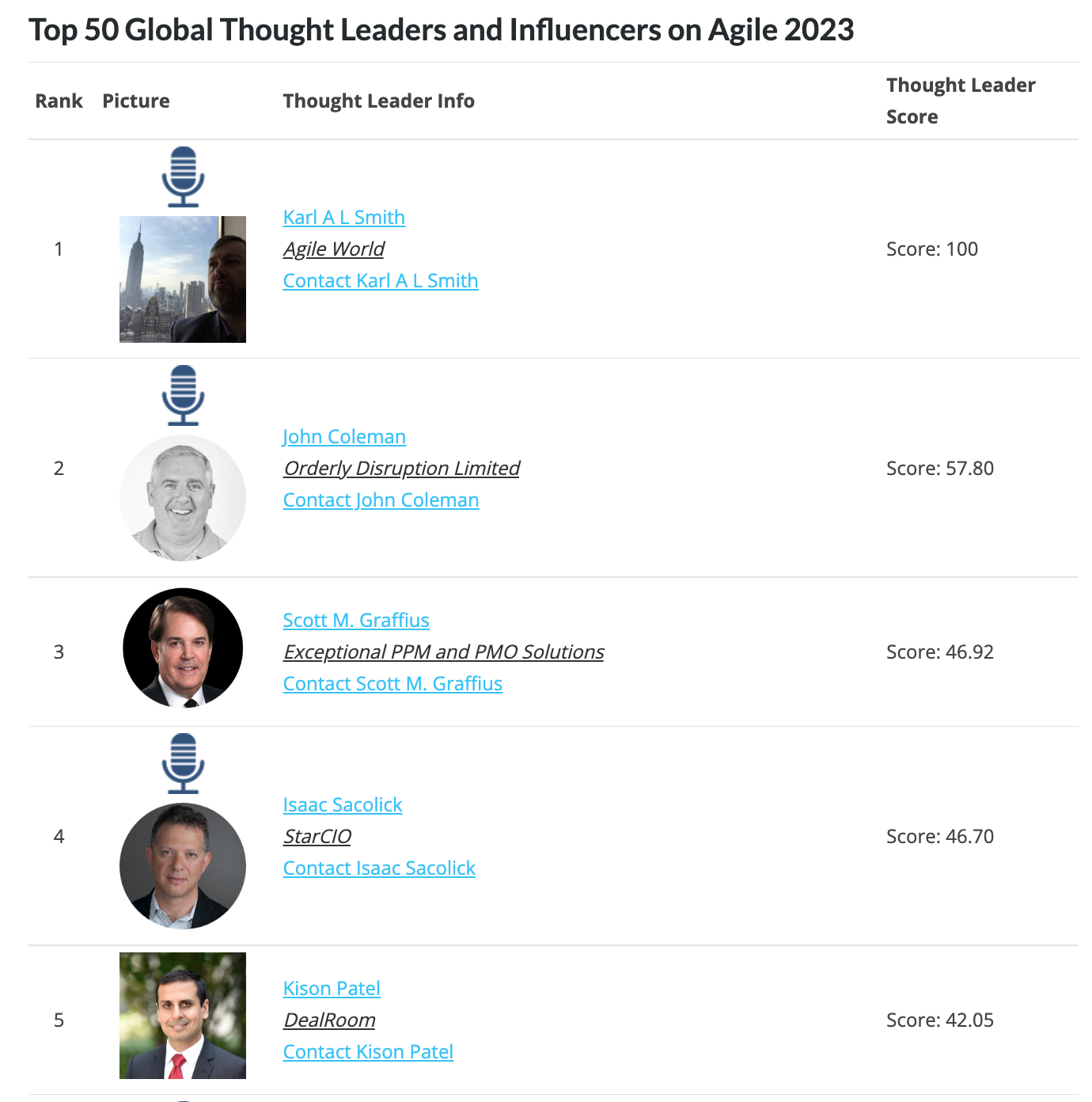The image depicts the profiles of five individuals recognized as top global thought leaders and influencers in Agile for 2023. The caption at the top reads, "Top 50 Global Thought Leaders and Influencers on Agile 2023" in bold black text. Below this title, a header categorizes the information into four columns: Rank, Picture, Thought Leader Info, and Thought Leader Score.

Ranked from 1 to 5, the images of these thought leaders are displayed with their corresponding numerical positions. Under the "Thought Leader Info" column, each row provides detailed information about the individuals, including their names, the companies they represent, and their contact details, which are underlined for emphasis. 

In the final column, "Thought Leader Score," the scores are listed as follows: the leader in the number one position holds a score of 100, the second position has a score of 57.80, the third has 46.92, the fourth 46.70, and the fifth holds a score of 42.05.